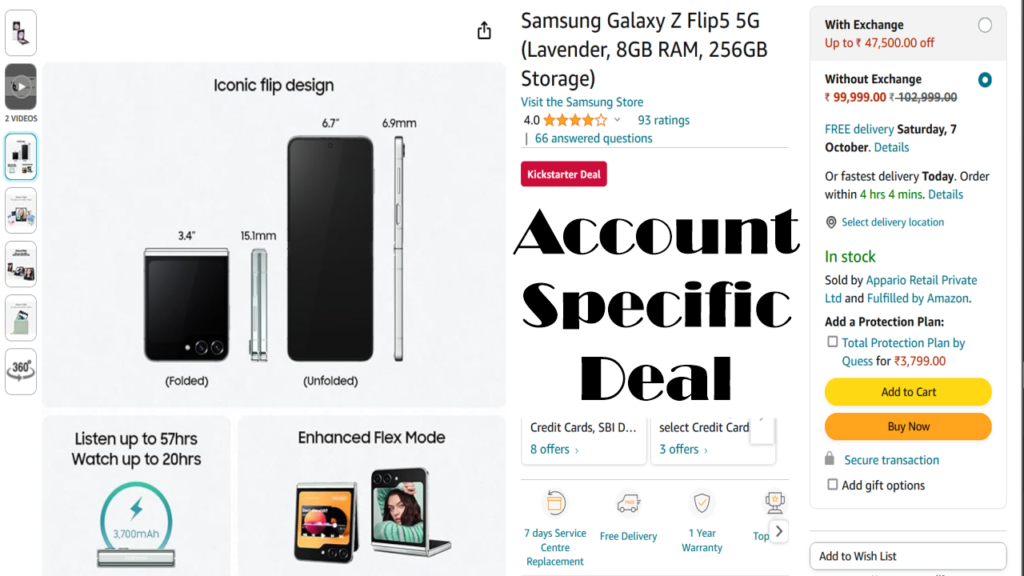Screenshot Description: 

The image is a screenshot of a product listing for the Samsung Galaxy Z Flip 5 5G on a retail website. The phone featured in the listing comes in a sleek lavender color and offers a configuration of 8GB of RAM and 256GB of internal storage. The product is available at the Samsung Store, where it has garnered a rating of four stars based on 93 customer reviews. 

There are various promotional offers available, including special discounts for certain credit card holders, a Kickstarter-specific deal, and up to a 7-day service center replacement policy. The phone is priced at what appears to be an equivalent of $99,999 in an unspecified currency, with an exchange offer that could reduce the price by up to $47,500 in the same currency. The listing guarantees free delivery by Saturday, October 7, or a faster delivery option available for orders placed within a specified time frame.

The product is listed as in stock, sold by FRO Retail Private LTD and fulfilled by Amazon. Moreover, a protection plan can be purchased for an additional $3,799. Several images of the phone are displayed, showcasing its unique flip design both when folded and unfolded. The device boasts impressive battery life, supporting up to 20 hours of video playback and 57 hours of audio listening on a single charge.